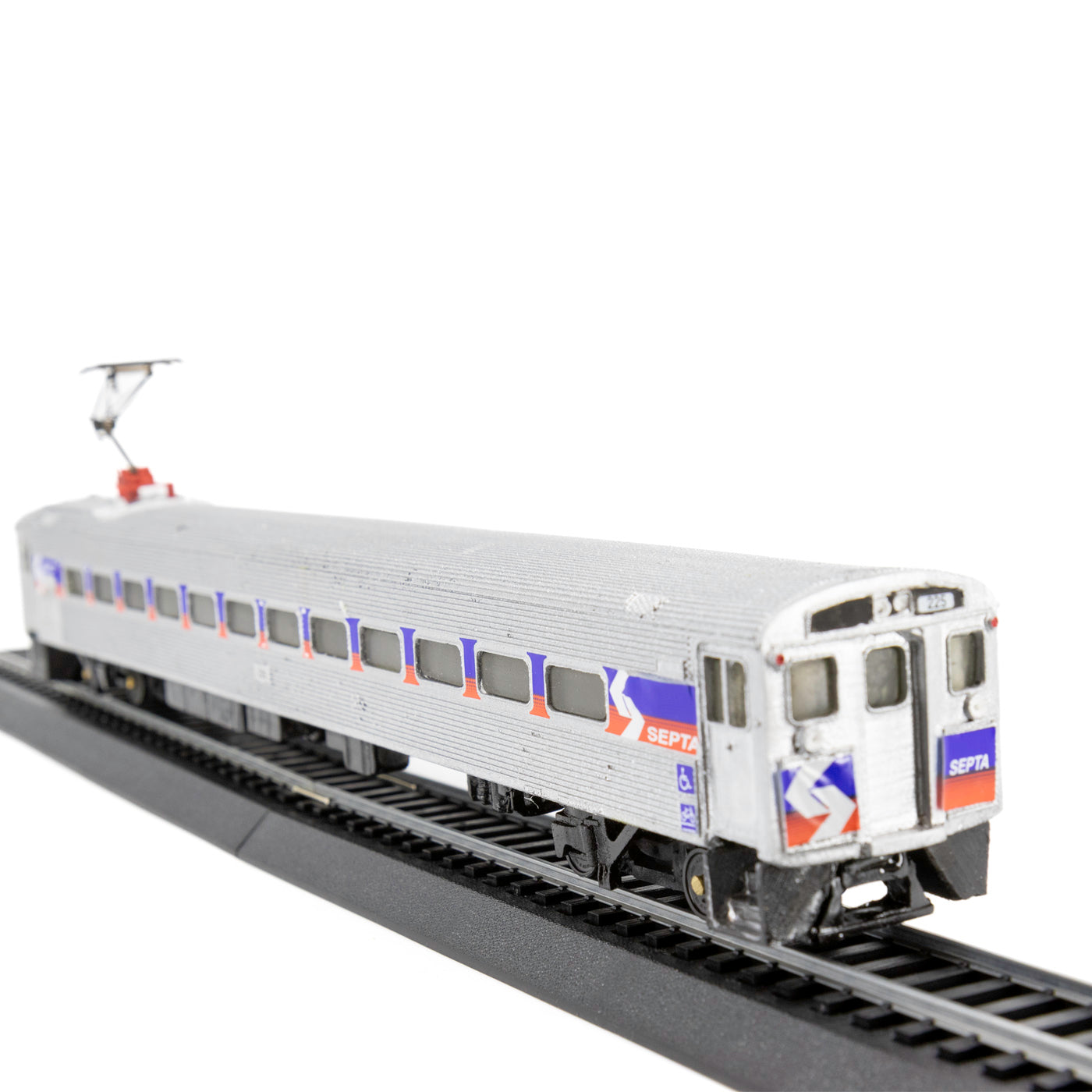The image depicts a detailed photograph of a miniature train car, seemingly a model or toy, captured against a completely white background. The black trapezoidal railroad bed runs diagonally from the bottom right corner of the image to the upper left, supporting black slats and gray rails. Atop the tracks sits a silver train car adorned with a blue and orange stripe pattern between each of its approximately 10 to 12 windows. Some windows have solid gray coverings, reinforcing the toy-like appearance. 

Prominently featured on both the front and side of the train car are signs with a white 'S' and the word "SEPTA," consistent with the Southeastern Pennsylvania Transportation Authority's logo. Near the front of the car is a white rectangle displaying the number "225." Additionally, there’s a red base at the back of the train's roof from which a T-shaped pantograph or armature extends, resembling a power connector device. The clarity of the train’s intricate details, combined with the contrast of the train against its monochromatic background, emphasizes the meticulous design of the miniature model.